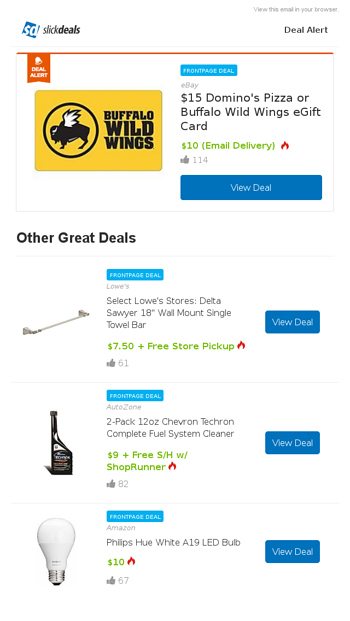The following is a detailed and cleaned-up caption for the given image:

In the top-left corner of the Slick Deals advertisement, a blue square with white "SD" initials is prominently displayed next to the site name "Slick Deals" in black, with "Deals" in bold. On the far right, bold black letters proclaim "Deal Alert," with the text "view this email in your browser" above in a gray font. An orange line separates this section from the content below.

Beneath the orange line, an orange flag icon featuring a white bell and the white text "Deal Alert" is shown. Below this, the image displays a significant deal featuring a Buffalo Wild Wings gift card. It reads: "Front Page Deal: eBay $15 Domino's Pizza or Buffalo Wild Wings e-Gift Card for $10 (Email Delivery)". A red fire icon denotes its hot status, accompanied by 114 thumbs-up likes and a prominent blue button with white text that reads "View Deal".

Following this, there's a "Front Page Deal" for Lowe's, showcasing a Delta Sawyer 18-inch wall mount single towel bar for $7.50 with free store pickup. Again, a red fire icon indicates its popularity, with 61 thumbs-up likes and a "View Deal" button in blue with white text.

Next, a "Front Page Deal" from AutoZone is highlighted, offering a two-pack of 12-ounce Chevron Techron complete fuel system cleaner for $9, including free shipping and handling with ShopRunner. This deal is marked with a red fire icon, has garnered 82 thumbs-up likes, and features the familiar blue "View Deal" button.

At the bottom, there's a deal from Amazon for a Philips Hue white A19 LED bulb priced at $10. This offer also bears the red fire icon and has 67 thumbs-up likes, along with the blue "View Deal" button.

This cleaned and detailed caption efficiently describes the contents and layout of the Slick Deals advertisement image.